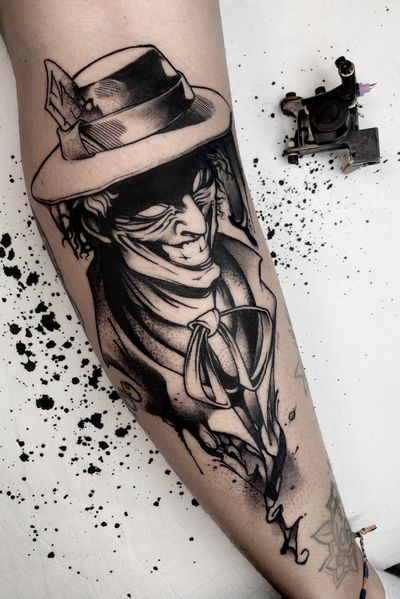This detailed color image captures the forearm of a woman as a new tattoo is being created. The arm is resting on a white surface splattered with black ink. Scattered around are pieces of tattoo equipment, including an ink pad positioned to the side and a tattoo gun laying flat. The freshly inked tattoo stretches from the inside of her elbow down to almost her wrist, depicting a sinister, Joker-like character whose face is adorned with a big smile revealing scary teeth. The character has a sharp jawline, a hooked nose, wide eyes, and is wearing a top hat along with a floppy bow tie. The tattoo is done entirely in shades of black ink, enhancing its dark, graphic novel or cartoon style. There is another faded tattoo near her wrist and a small, almost indiscernible tattoo along with a white sock and an ankle bracelet on her ankle. The meticulous detail in the new tattoo, combined with the ongoing inking process, lends the image a dynamic and eerie atmosphere.